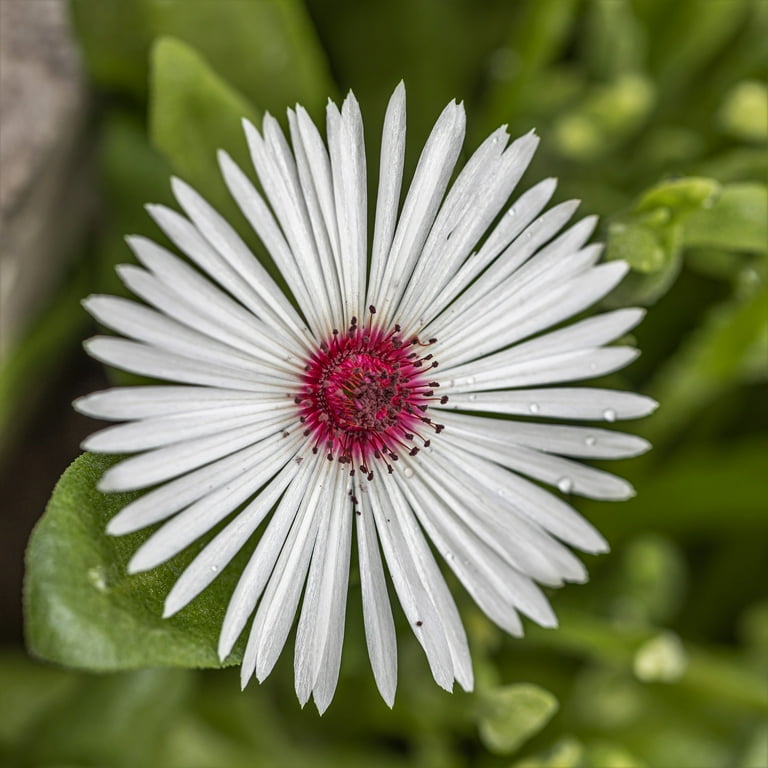This close-up macro shot captures a stunning white flower, reminiscent of a daisy, with numerous long and thin petals radiating outward. At the heart of the flower lies a vibrant, hot pink center adorned with delicate, furry stamen-like structures that vary in shades of pink and burgundy. The meticulous focus on the flower reveals exquisite details, including a few tiny, glistening water droplets on the petals. The background, enveloped in a lush green blur, hints at surrounding foliage with an indistinct gray rock peeking in from the upper left corner, adding texture to the soft, dreamy backdrop. The contrast between the sharply defined flower and the softly blurred surroundings emphasizes the flower's delicate beauty.